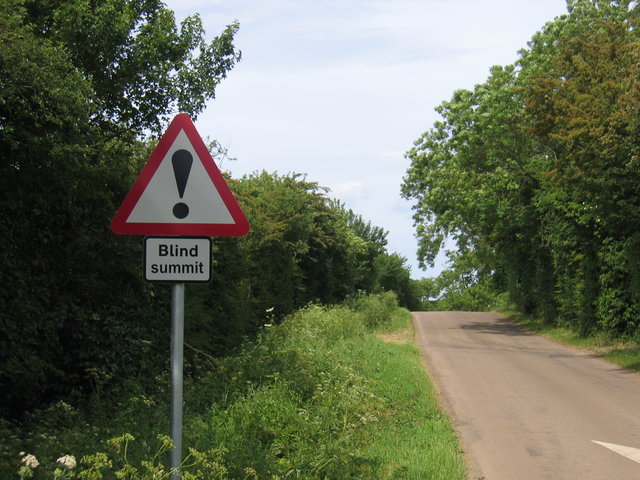This is an outdoor photograph, likely taken by a pedestrian, featuring a narrow, grayish dirt or slightly paved road curving from the bottom right into the distance toward the middle right of the image, seemingly leading downhill. The setting is a lush forest with vibrant shades of green, ranging from trees to shrubs, and wildflowers interspersed with bushes. To the left of the road, the greenery appears more natural and untamed, featuring an array of wildflowers, while the right side shows more orderly, trimmed trees. 

Central in the image is a prominent road sign: a red-outlined, white triangular sign with a black exclamation mark in its center, mounted on a pole. Beneath it, a smaller white sign reads "Blind Summit," indicating a bump in the road that obscures oncoming traffic. The sky above is mostly cloudy with patches of blue visible, suggesting it is a predominantly overcast day. The scene is devoid of any human presence, exuding a serene and undisturbed atmosphere.